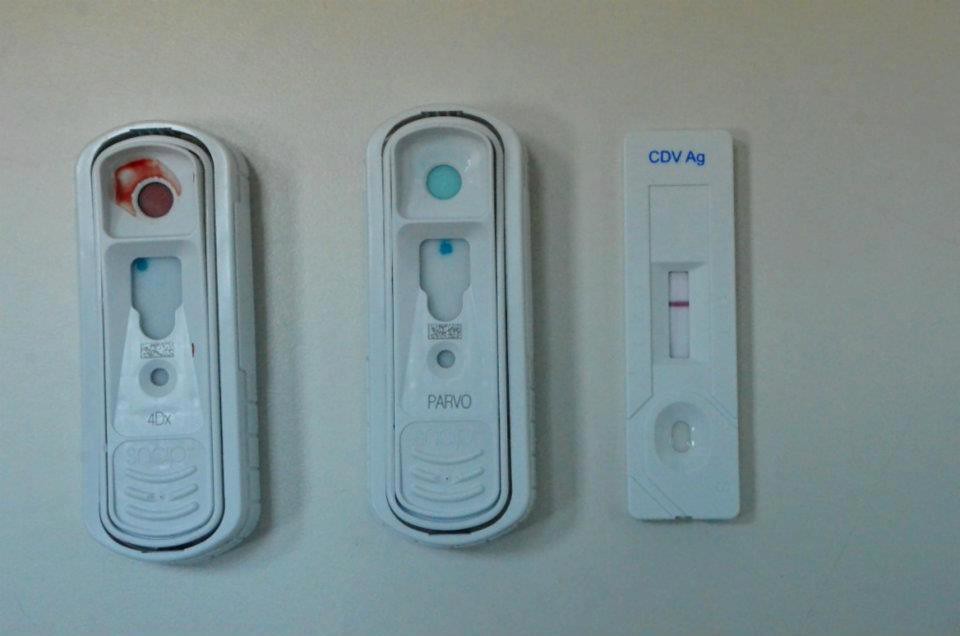The image showcases three distinct types of test strips arranged side by side. Starting from the left, the first two test strips feature an oblong, rounded design with a small window displaying the test results. The test strip on the far left has a red coloration at the top, indicating the area where the sample, possibly blood, is applied. In its window, a reddish hue suggests that it might be conducting a blood-related test. The strip in the center has a clear, blue-toned window, which might imply that it is designed to test a different substance or parameter. On the right, the third test strip diverges in shape, adopting a more squared form. It includes a distinct viewing window for observing the test results and an indentation where the test sample, potentially a liquid or bodily fluid, is deposited.